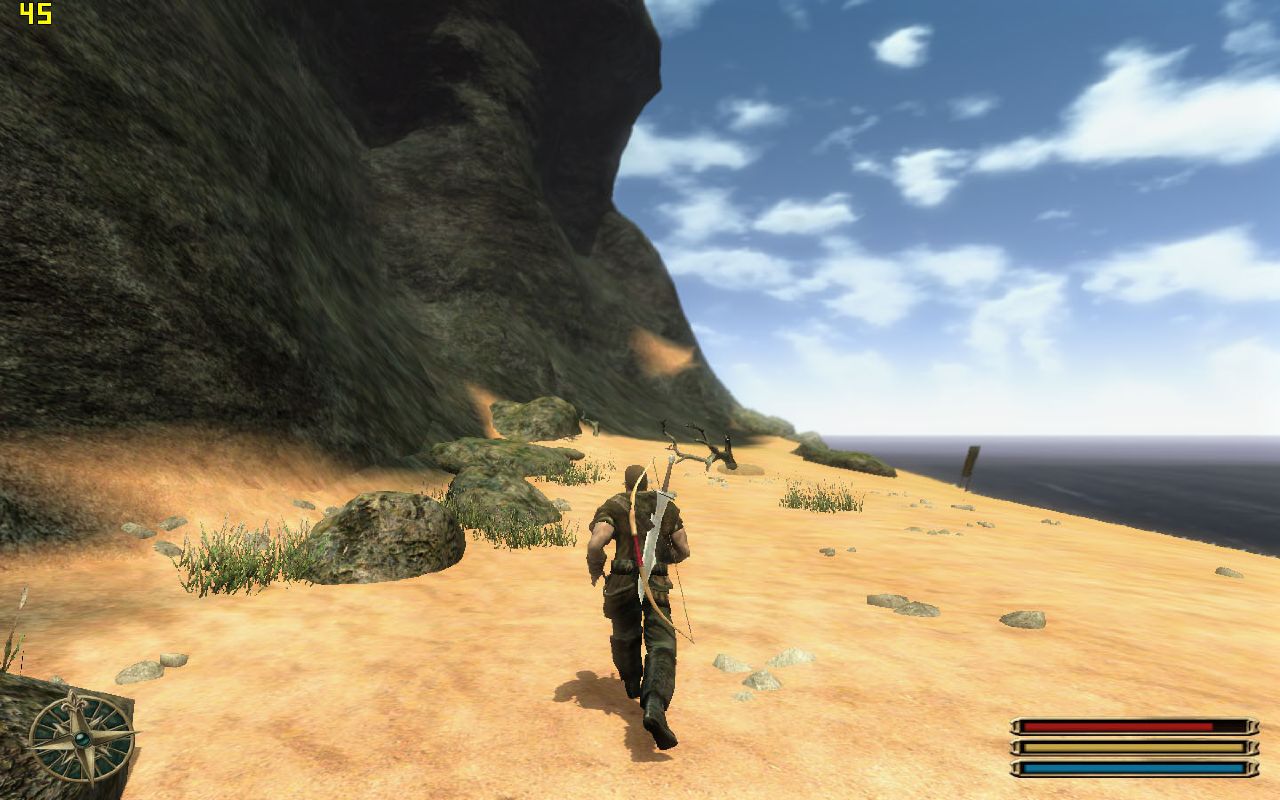A detailed screenshot from a computer game captures the back of a male character traversing a sandy beach. The character is equipped with a long sword slung over his right shoulder and a bow featuring a striking red handle, indicating his readiness for combat. In the bottom left corner of the screen, a compass icon aids in navigation. To the right, three horizontal bars display various in-game statistics: a full blue bar at the bottom, a fully charged yellow bar in the middle, and a red bar, likely representing health, which is approximately 80% filled. The scene is set against an expansive beach flanked by towering cliffs on the left and the vast ocean on the right. The sky above is vibrant blue, dotted with numerous white clouds, enhancing the scenic view. The character's attire consists of a rugged brown outfit with short sleeves and sturdy boots, fitting for an adventurer in this dynamic environment.